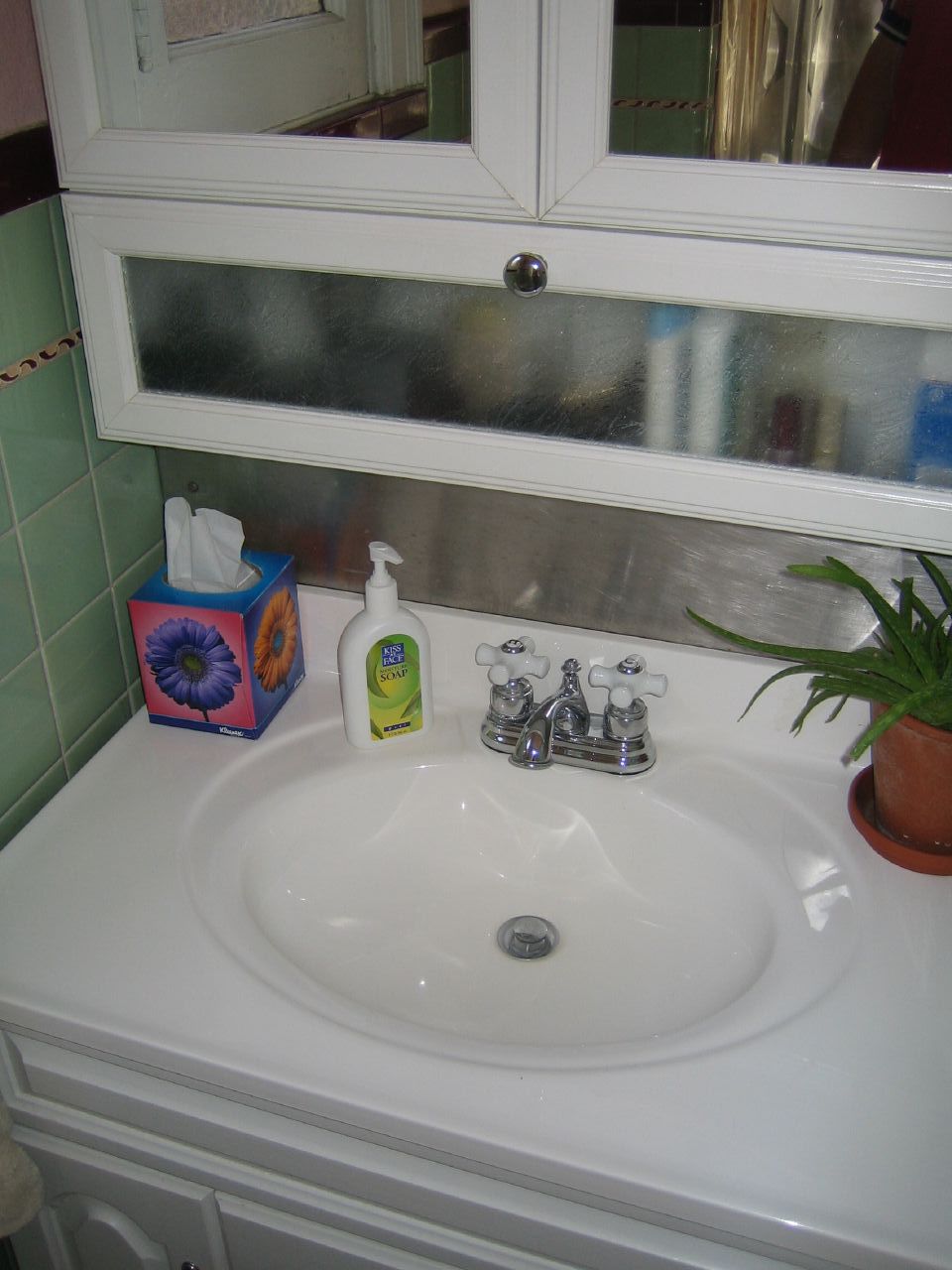In this tilted photograph of a bathroom, likely taken accidentally with a cell phone at a 45-degree angle to the right, a myriad of details can be observed despite the haphazard composition. Dominating the scene is a clean, white countertop hosting a white sink with twin silver faucets, each featuring separate hot and cold knobs. Atop the counter, on the left, rests a blue Kleenex box adorned with purple and orange floral patterns. Beside it, a green and white hand soap bottle stands for easy access. Adding a touch of nature, an aloe plant or a similar succulent is potted in a terracotta planter with a matching dish. Above the sink, on the right side of the image, a white mirrored cabinet offers both reflective surfaces and a frosted glass section. The frosted glass obscures but reveals a hint of the stored items behind it, adding a slight element of mystery to this ordinary yet visually busy bathroom scene.